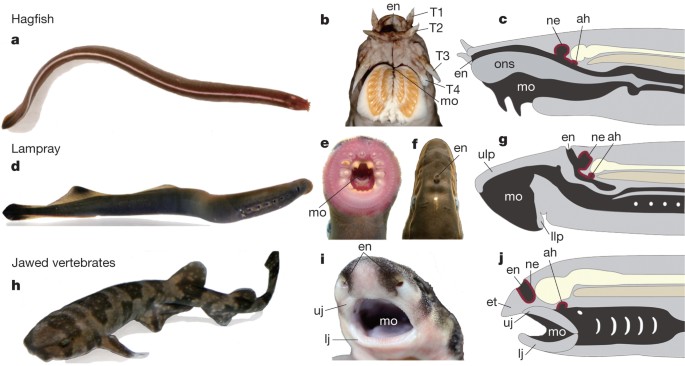This detailed diagram on a white background showcases various oceanic creatures, specifically a hagfish, a lamprey, and a juvenile shark, capturing both photographic and illustrative representations. 

On the left, the diagram features:
1. **Hagfish** (labeled "A") - an eel-like creature, brown with a white underside and stripe, followed by a close-up illustrating its anatomical features. Additionally, the underside jaw labeled "T4" and feelers "T1, T2, T3" with the mouth marked as "B".
2. **Lamprey** (labeled "D") - a dark brown creature resembling an eel, characterized by its circular tooth-lined mouth. Accompanying this is a detailed view of its mouth labeled "MO" and sections indicated as "EN".
3. **Jawed Vertebrates** (labeled "H") - a small juvenile shark with distinctive spots, showing sensory organ highlights such as "EN" for the nose, "MO" for the mouth, "UJ" for the upper jaw, and "LJ" for the lower jaw.

Central to the image are additional detailed diagrams:
- **Hagfish Jaw**: Detailed anatomical labels including "EN" for the top, and various teeth and underside parts marked.
- **Lamprey Mouth**: A close-up of its distinct teeth arrangement labeled "MO" and the end marked as "EN".
- **Shark Anatomy**: Showcasing mouth and sensory parts, with differing labels "EN, MO, UJ, LJ".

On the far right, illustrative diagrams succinctly represent these creatures with internal structures:
- **Hagfish (C)**: Labeled with parts like "NE, AH, ONS, MO, EN".
- **Lamprey (G)**: Detailed labels from "EN, NE, AH, LLP, MO, ULP".
- **Juvenile Shark (J)**: Featuring label sequence "AH, MO, LJ, UJ, ET, EN, NE".

The overall structure follows three vertical columns, juxtaposing realistic photography with schematically labeled drawings to illustrate the intricate anatomy of these fascinating marine beings.